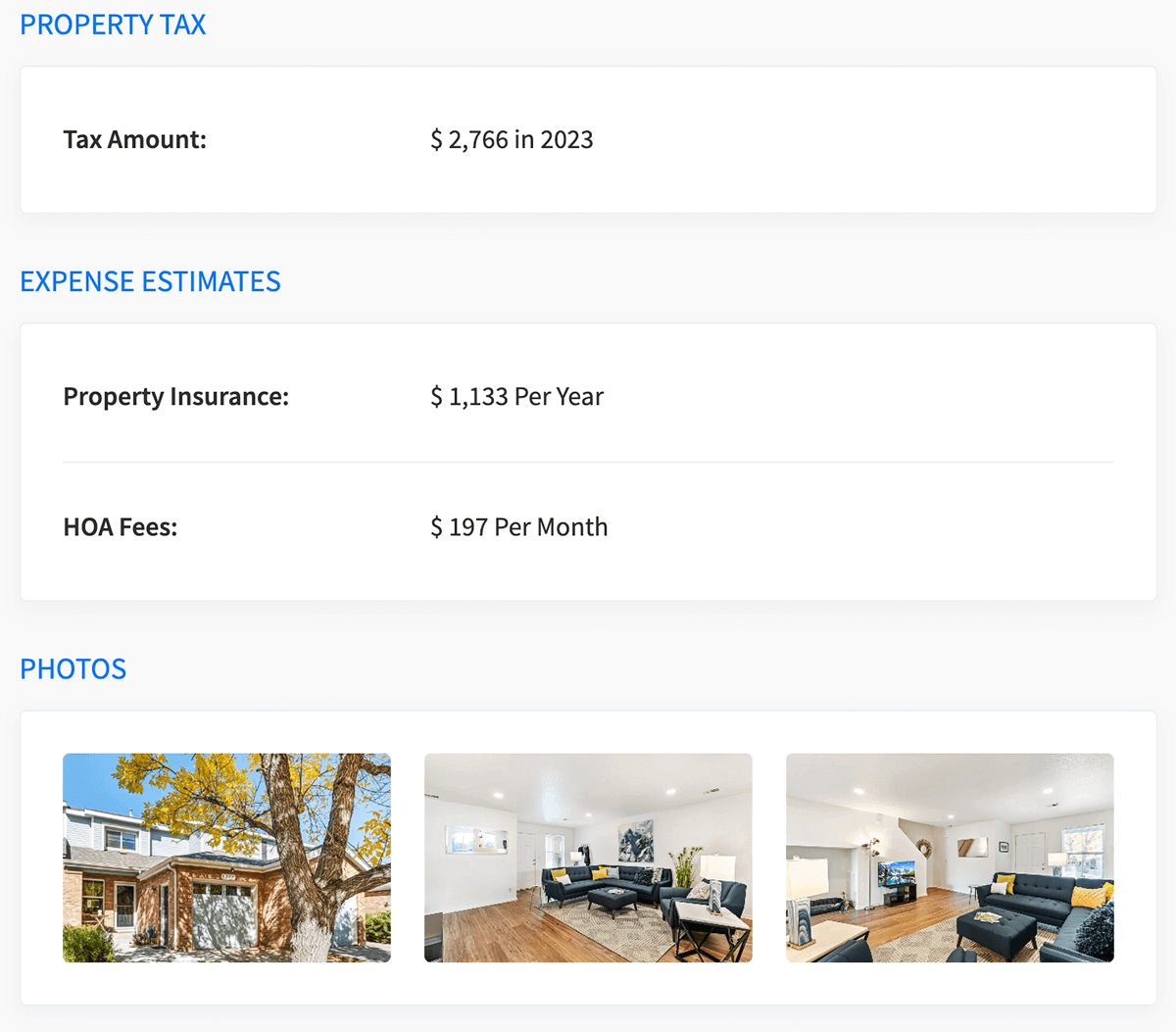The image features a detailed real estate property advertisement on a white background. At the top, a shaded banner stretches horizontally, displaying the text "Property Tax" in blue on the left side. Below it, a white banner spans the width of the image, with the caption "Tax Amount: $2,766 in 2013" positioned centrally.

Continuing downward, there's another shaded section on the left with the label "Expense Estimates." Adjacent to this, a white banner details various costs: "Property Insurance: $1,133 per year" and "HOA Fees: $197 per month."

On the left side again, there is a section labeled "Photos," which showcases three images of the property. The first photo depicts a two-story home with a large tree in the front yard. The upper portion of the home is white, featuring a sizable window, with a white garage door on the right and a white front entrance. The house is composed of a blonde brick facade, complemented by shrubbery in the front yard.

The second image highlights a living room with brown wooden floors, a black leather sofa and chair, and black coffee tables. The room is accentuated by white walls and built-in ceiling lights.

The third photo continues to feature the living room from a different perspective, showcasing the black sofa, coffee tables, and a staircase ascending to the next level. This angle also reveals a flat-screen TV mounted against the wall, the front door, a front-facing window, and a large throw rug situated in front of the sofa.